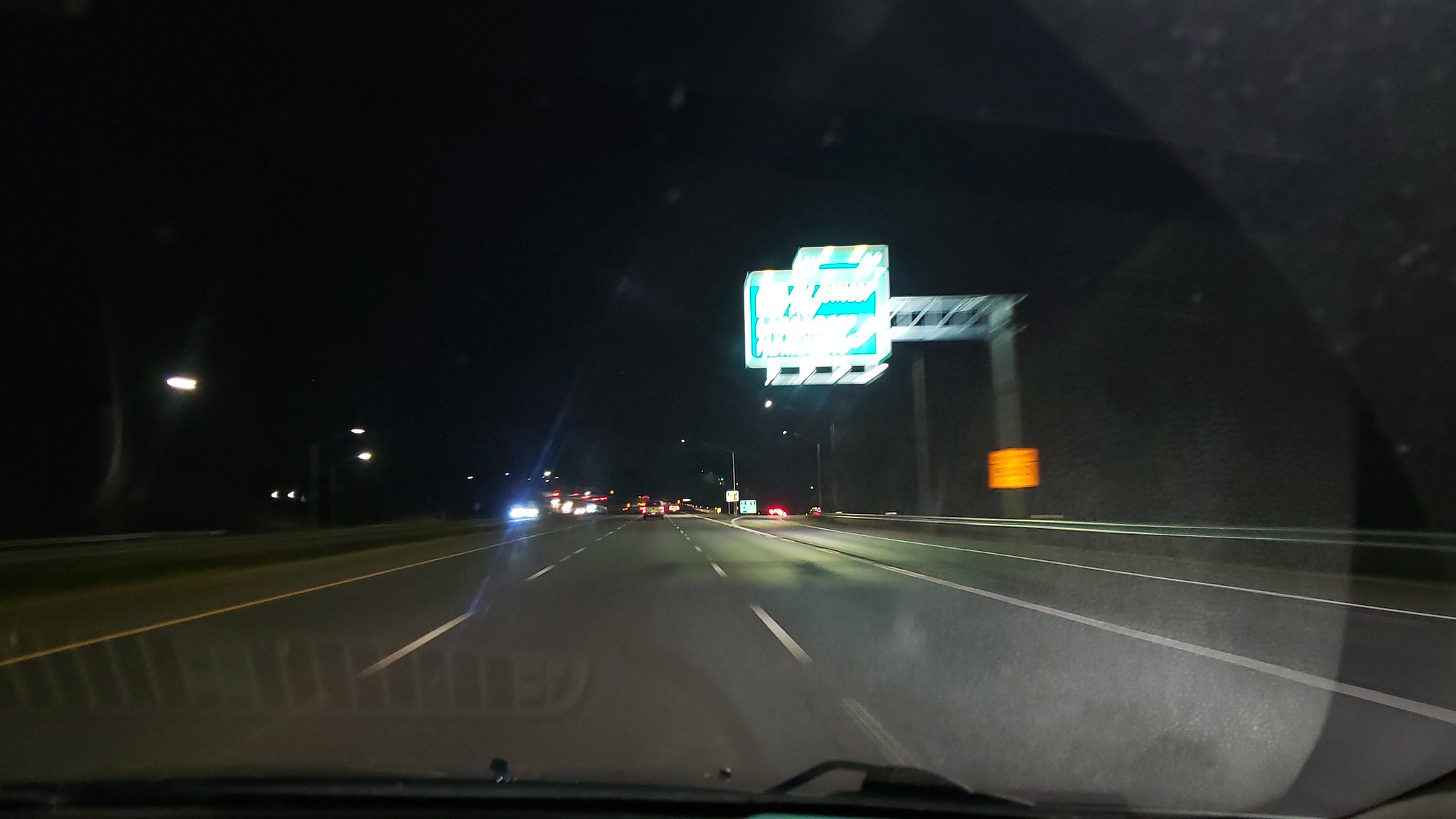The photograph captures a nighttime highway scene, shot through the windshield from a passenger’s perspective. The bottom edge of the image shows a fragment of the dashboard and the folded windshield wipers. The highway, appearing nearly empty, stretches ahead under a black sky devoid of stars. A few scattered streetlights line the left side of the road, while the right side features an exit ramp marked by red car taillights. Oncoming traffic consists of a few distant car headlights. A large green highway sign hangs blurry and unreadable near the center-top of the image. The photo suggests motion, indicated by the overall blur and the smudge of dirt in the upper right corner, possibly tracing the wipers' path. Dotted white lane markers define the road lanes, and the perspective implies the car is traveling in the middle lane.